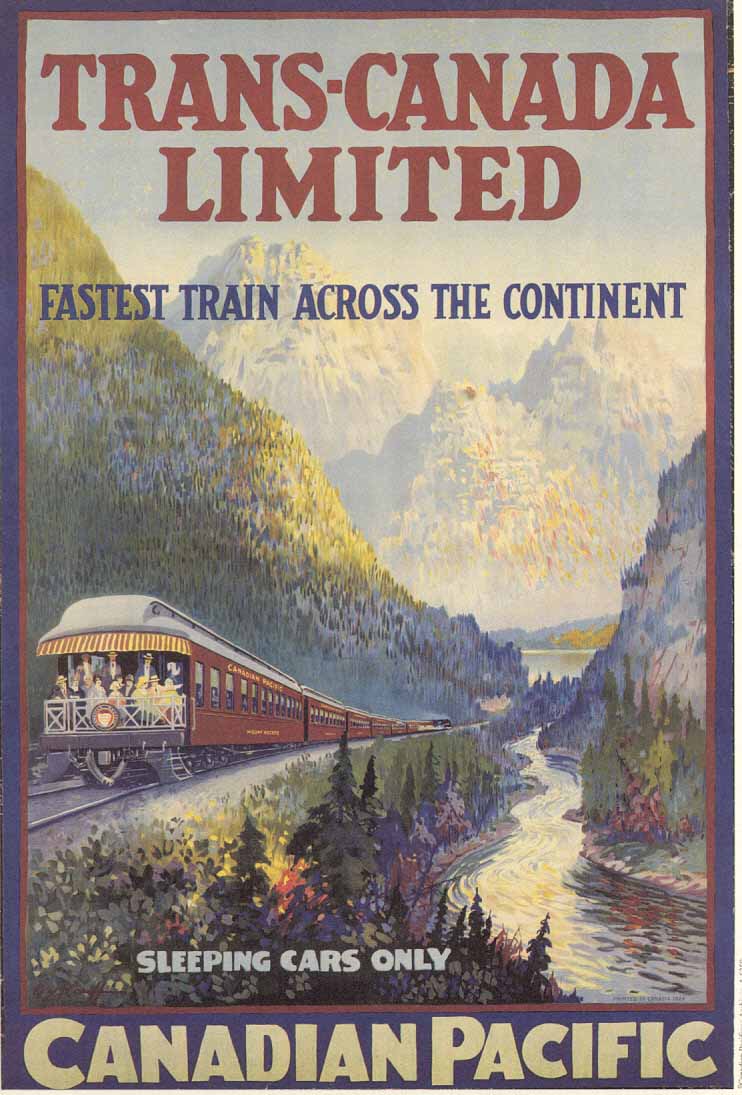This vintage advertisement for Canadian Pacific Railroad's Trans-Canada Limited showcases the fastest train across the continent, dedicated solely to sleeping cars. The painted image captures a scenic journey through nature, with the red passenger train prominently featured in the lower part of the blue poster, bordered in red. Passengers can be seen standing on the caboose, gazing at the majestic landscape. The train travels beside a winding river surrounded by lush greenery, and in the background, steep, rocky mountains rise, some possibly snow-capped. The poster highlights the elegance and speed of the train, with bold red and blue letters proclaiming its name and distinction as the continent's fastest train. The poster includes the tagline "Sleeping Cars Only" and proudly features "Canadian Pacific" in white letters at the bottom.